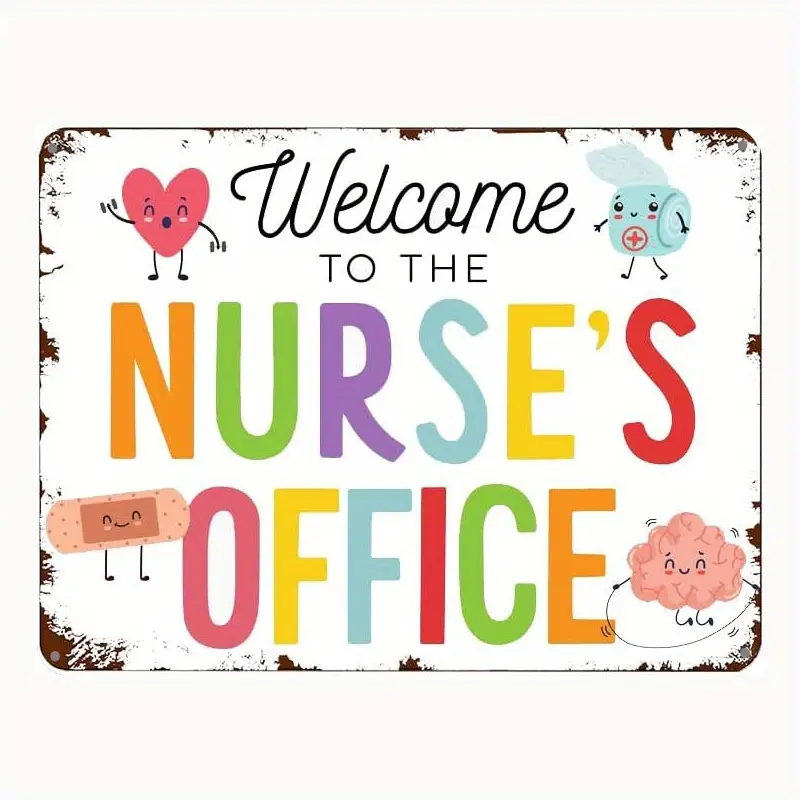The image features a photograph of a white poster that shows deliberate wear and tear, giving it a vintage feel with worn paint edges. At the top of the poster, "Welcome to the" is written in elegant cursive script, followed by "nurse's office" displayed in vibrant, rainbow-colored letters. Each letter in "nurse's office" is uniquely colored to create a cheerful rainbow effect. 

In the top-left corner of the poster, there is a heart character lifting dumbbells, symbolizing strength and health. The top-right corner features a smiling bandage, adding to the friendly and welcoming atmosphere. In the bottom-left corner, a small, cheerful band-aid character can be seen, while the bottom-right corner showcases a brain character engaging in jump rope exercise, radiating a sense of fun and activity.

This inviting and playful sign, likely intended for a school nurse's office, exudes warmth and cheerfulness, making it an ideal decoration to make anyone visiting feel safe and comforted.